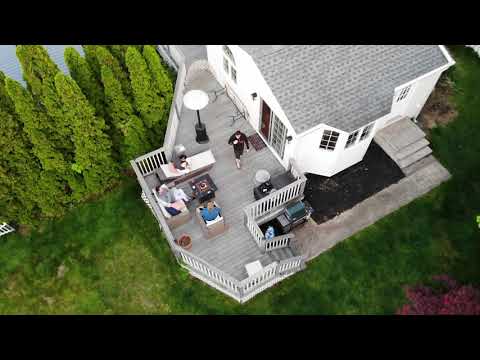The image captures an overhead view of a white house with a grey roof, set in a lush green landscape. This aerial perspective highlights a detailed patio connected to the home, featuring white railings and a sliding door. The patio, which is situated on the second floor, includes a love seat, a small couch, a table, and a lamp. Several people are gathered on the patio, with one individual in a blue shirt looking directly up at the drone. The stairs from the patio lead down to a walkway bordered by greenery. The backyard shows vibrant green grass, with a purple pile of leaves or similar located in the bottom right corner. The setting is an outdoor daytime scene, possibly overcast due to minimal shadows. Trees are visible at the top left and right of the image, adding to the tranquil atmosphere.